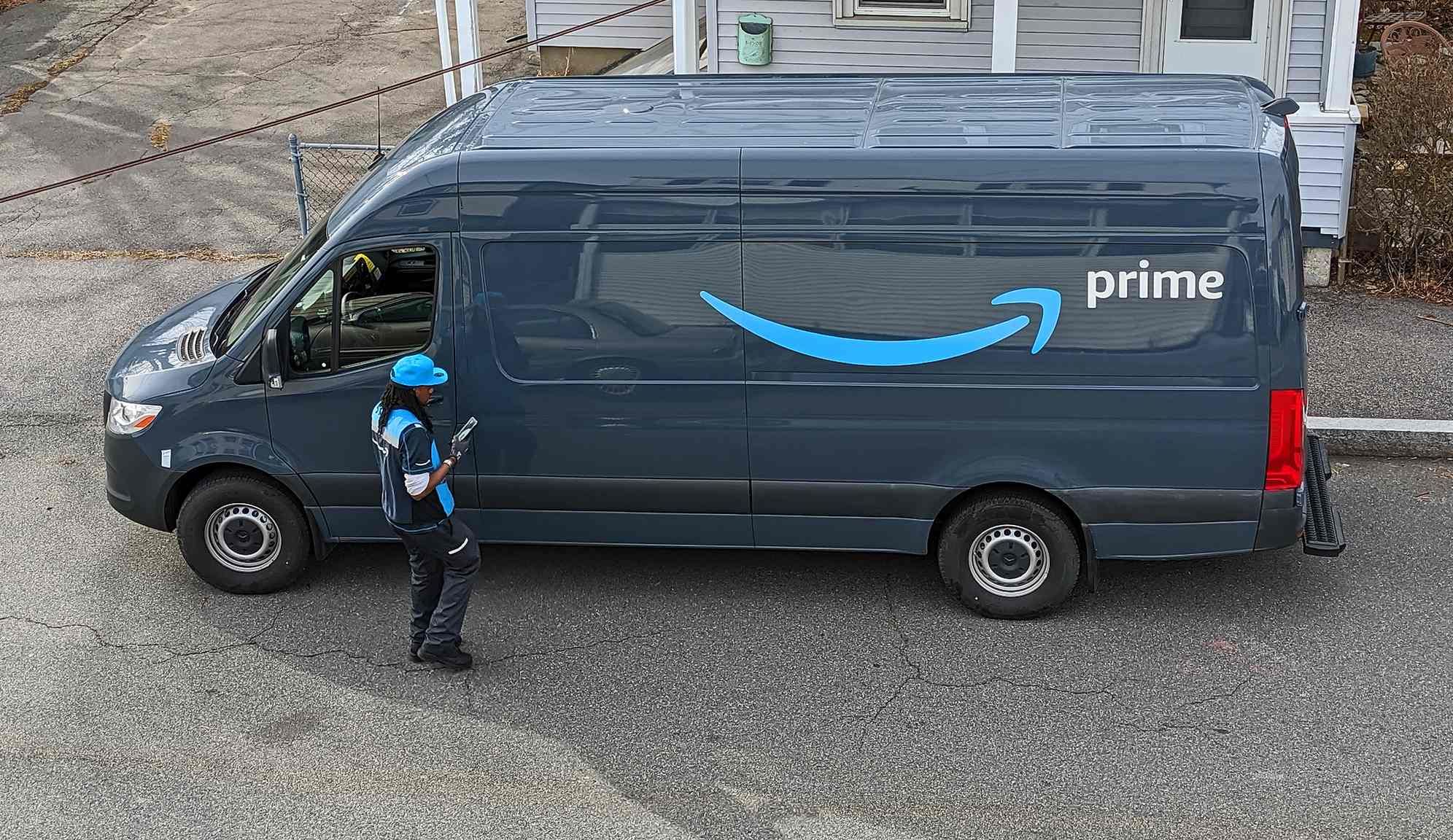A gray Amazon Prime delivery van, featuring the iconic Amazon arrow logo on its side, is parked outside a classic American-style wooden home with white planks. An Amazon employee stands just outside the driver's door, dressed in a coordinated outfit comprising gray trousers and a gray T-shirt with a distinctive blue stripe that echoes the van's branding. The individual, likely female due to her long hair, appears to be checking her phone, possibly to confirm delivery details. The spacious van, equipped with a small tailgate at the rear for easier access, has its driver's window rolled down, indicating a quick stop. The scene is set at a junction in a residential neighborhood, adding to the quintessentially American atmosphere.